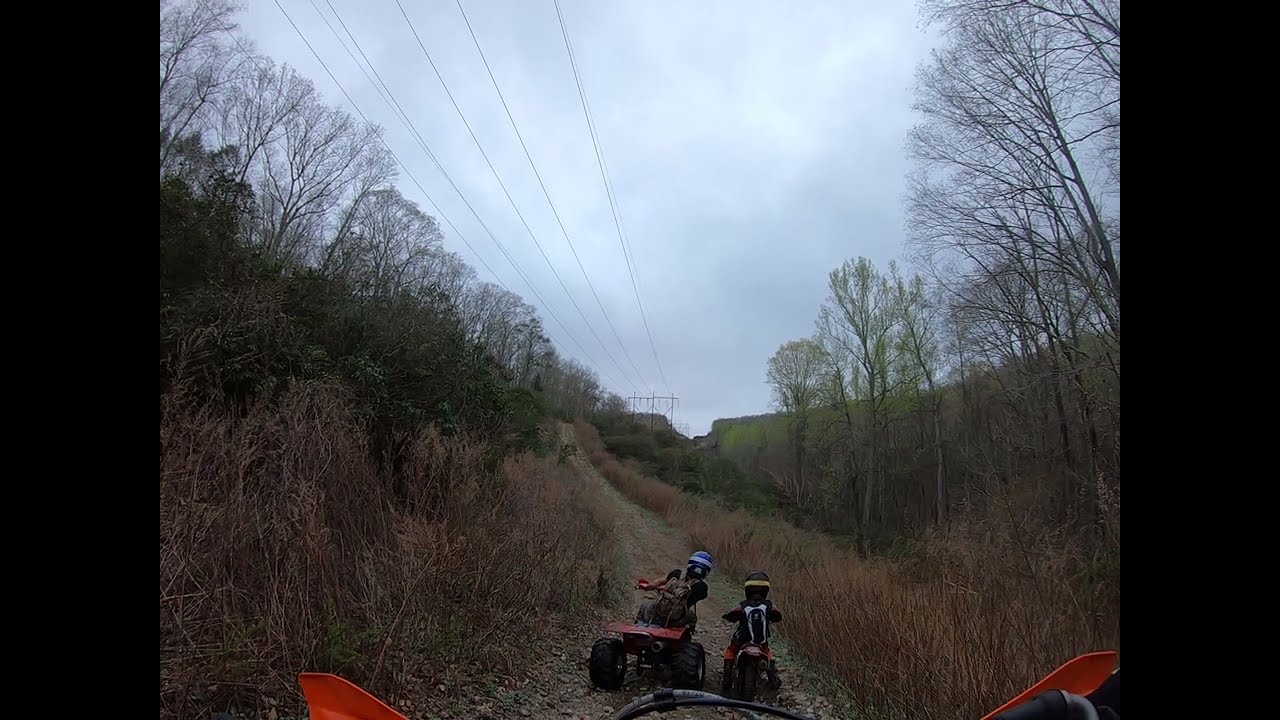In this outdoor image taken during the daytime under a sky filled with gray clouds, we see a scenic dirt trail flanked by a mix of bare and green-leaved trees, along with patches of dry, dead weeds and large grass. The image captures an adventure featuring two children riding off-road vehicles; one child on a quad to the left dons a helmet and carries a backpack, while the other child on a small dirt bike to the right also wears a helmet. They are navigating the rocky trail, which is adorned with power lines stretching towards a distant metal structure. The setting displays a blend of earthy tones and vibrant colors, including blue, white, gray, black, green, orange, and red. All the elements converge in the lower center of the frame, providing a captivating snapshot of nature and youthful exploration.